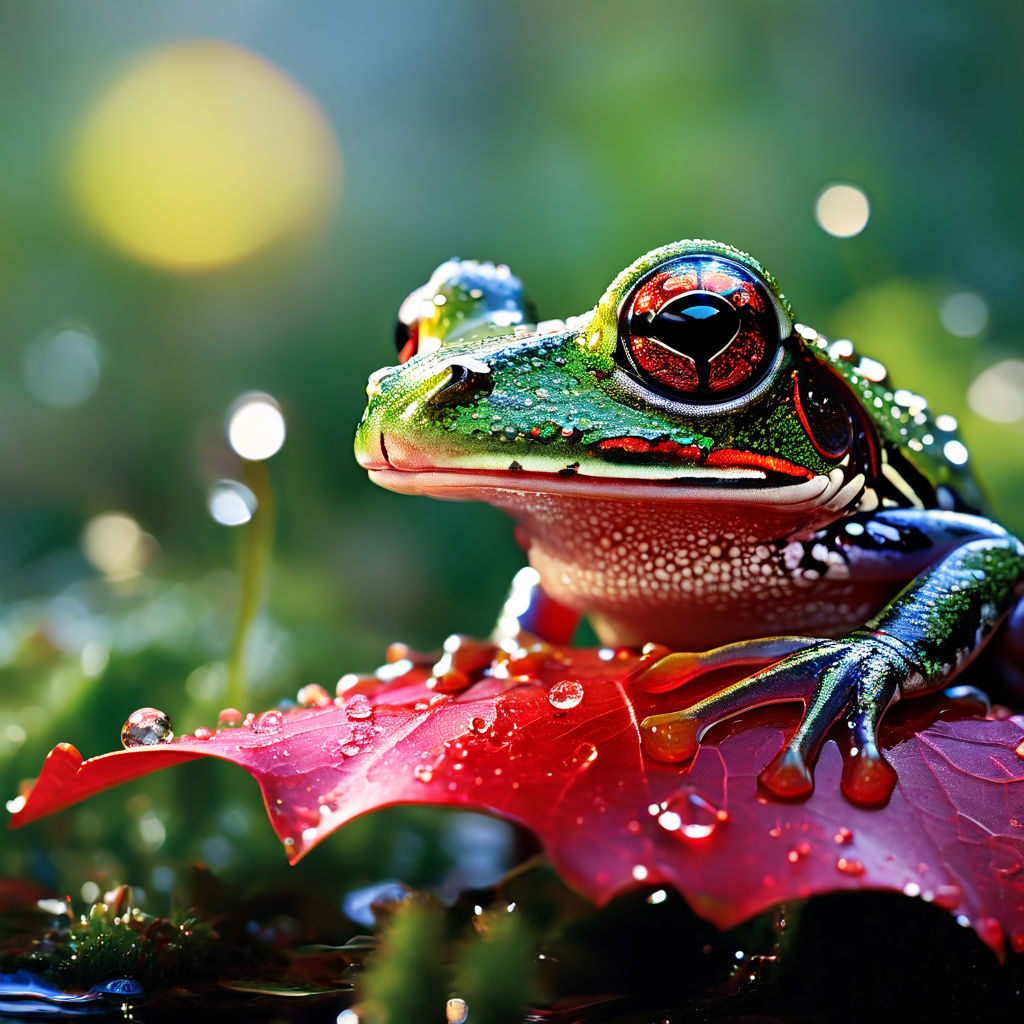The image is a highly detailed, professional photograph showcasing a vividly colored frog perched on a bright red leaf. The frog's body is predominantly green, with large, bulging red eyes featuring black pupils. Its front legs and four fingers, which have distinctive red dots, are visible, while the rest of its legs are folded underneath its body. The frog's underside is a yellowish white, contrasting with its green top adorned with water droplets. The leaf it rests on is also studded with dew, adding to the realism of the scene. The background is intentionally blurred, emphasizing the frog and the leaf, and consists of green plants and a possible body of water, suggesting a natural habitat such as a pond or a marsh. A blurred yellow circle in the upper left corner hints at the sun, contributing to the overall immersive and lifelike quality of the image.